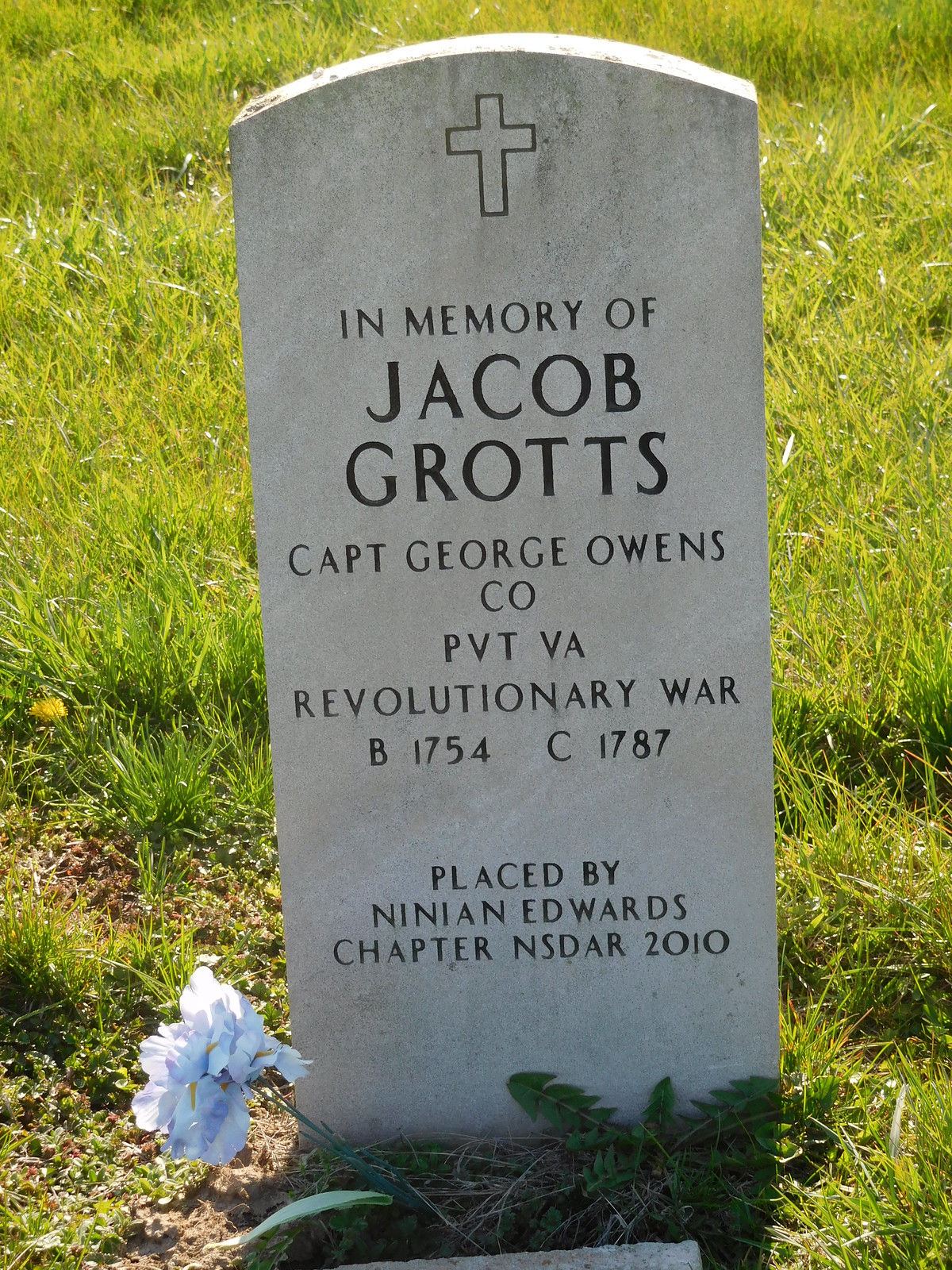The photograph, taken during the daytime, captures a serene cemetery scene dominated by a prominent headstone. The headstone, made of gray granite, stands upright about three times as tall as it is wide with a slightly curved top. At the very top of the gravestone, an etched cross is visible, symbolizing faith. In front of the gravestone, a vibrant blue-petaled flower with a green stem lies nestled in the lush green grass. The engraving on the gravestone reads, "In memory of Jacob Grotz, Captain George Owens Company, Private VA, Revolutionary War, B. 1754, C. 1787." Additionally, it notes that the gravestone was placed by the Ninian Edwards chapter of the NSDAR in 2010. This headstone commemorates Jacob Grotz, who fought and died during the Revolutionary War.